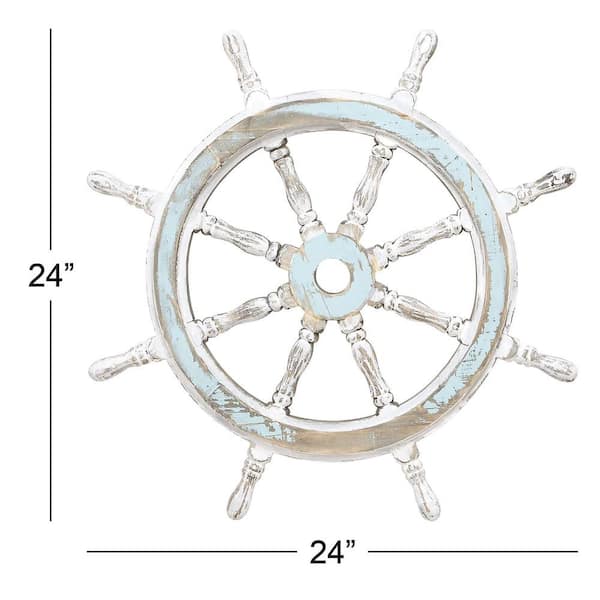This image is a detailed stock photograph of a vintage-style ship’s wheel, crafted from wood. The wheel has been painted a light aqua blue with sections of white, giving it a rustic, weathered appearance. Some of the white paint has been intentionally sanded away, revealing the aqua blue underneath, while parts of the blue paint have also been sanded to expose the pale wood beneath. The circular wheel features wooden knobs protruding around its circumference, resembling those on an old-time captain's steering wheel. Notably, the image includes measurement lines alongside and below the wheel, indicating that the piece measures 24 inches in both height and width, providing an exact scale of 24 by 24 inches.